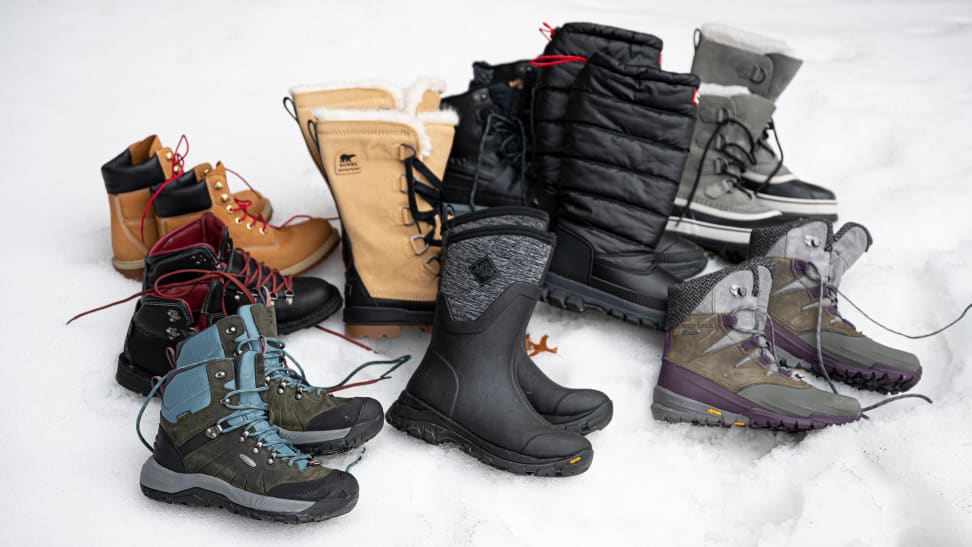This is a detailed image of nine pairs of winter boots, prominently displayed on a snowy white background. Each pair is arranged slightly on its side with one boot closer to the camera. The image depicts a variety of styles specifically designed for cold, snowy weather, offering a glimpse into different levels of insulation and waterproofing.

In the very center, there's a prominent black rubber pair, flanked by a tan fur-lined pair behind it and a sturdy black pair with a down-like material and red straps. To the right of the black rubber boots is another thick black pair, and further to the right, a pair of heavy gray boots with white fur trim. Clustered towards the front center-right is a pair of brown, purple, and gray lace-up boots. To the front center-left lies a distinctive blue and green pair. Behind these are a pair of black boots with striking red shoelaces and a pair of brown boots with black detailing and red laces adjacent to them.

Each pair varies in height from ankle to mid-calf, showcasing different materials such as suede, leather, and rubber, exemplifying the diverse styles of winter footwear, ranging from classic lace-ups to easy slip-ons. The setting on a pure snow blanket emphasizes their functionality and design for harsh weather conditions.